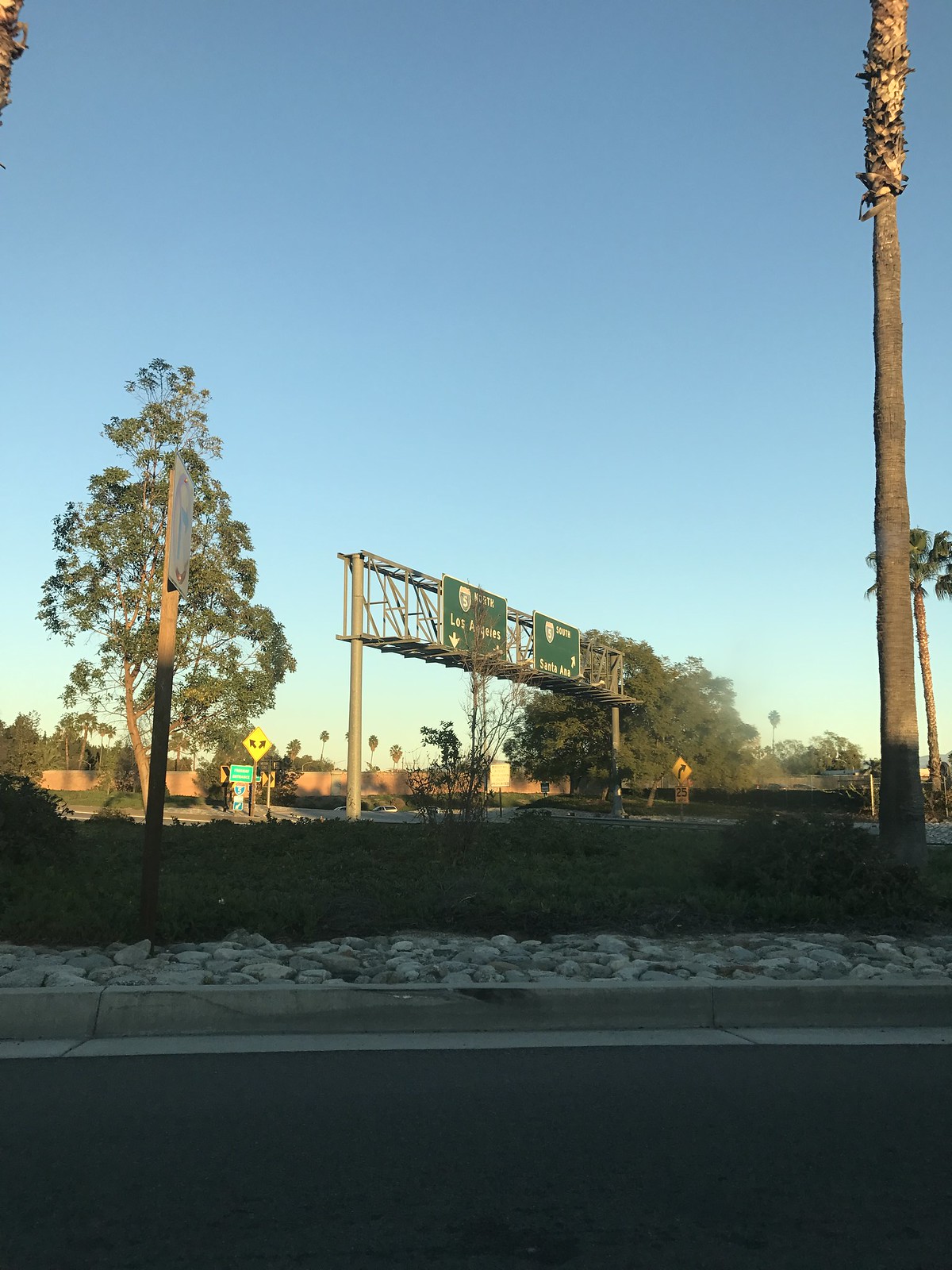The photograph captures a late afternoon scene of a freeway area, with the bottom third of the image cast in shadow and a vast, blue sky dominating the top portion. A hint of smog is visible near the horizon, giving the skyline a beige-ish tint. Distant palm trees dot the background, contributing to the characteristic Southern Californian landscape.

In the foreground, the trunk of a palm tree is prominently featured, though its top is out of frame. To the left, a larger deciduous tree adds greenery to the scene. A small section of street is visible, leading to a stone pathway, a meticulously trimmed hedge, and a traffic sign indicating no right turn. 

Behind this, the freeway comes into view, accompanied by a large directional sign displaying "5 North Los Angeles" with two arrows pointing downward, and another sign hinting at "3 North Santa Ana" with an arrow marking an off-ramp. Additional signs delineate various freeway routes and intersections.

The street itself is not visible, but the surrounding elements vividly depict the bustling infrastructure and natural beauty typical of this urban setting.